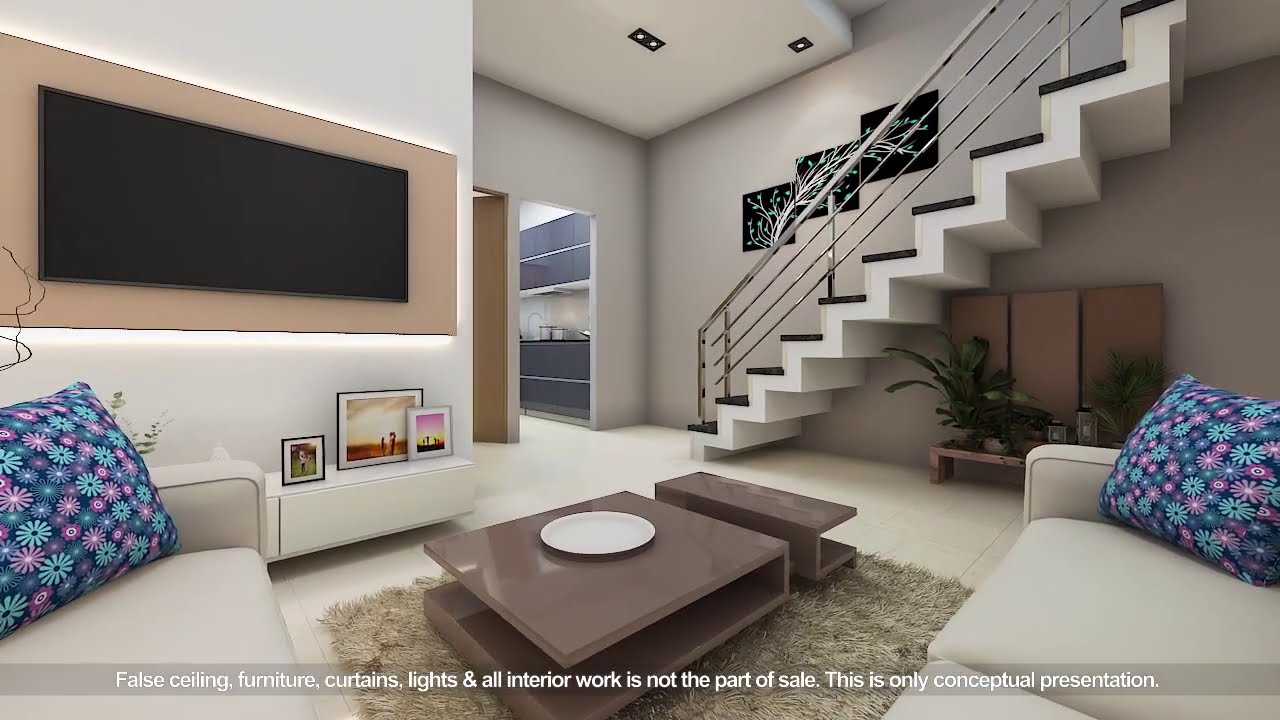The image depicts a meticulously designed and modern condominium interior, captured in vivid color. At the center, a furry, light brown floor mat is seen, adorned with an elongated, square-shaped dark brown table featuring a single white plate. Flanking the scene are beige sofas with cushions that showcase blue, purple, and pink floral patterns. On the left side, a white stand holding three picture frames sits beneath a large black space intended for a widescreen TV.

A series of sleek, chrome-handle staircases ascend towards the upper floor, accompanied by various plants on a nearby round stand. To the right of the stairs, an open doorway reveals an organized kitchen with black cabinets and gray countertops. The overall aesthetic is completed by white walls adorned with flower-themed art, creating a clean, vibrant, and welcoming atmosphere. Notably, a caption on the bottom of the image reads, "False ceiling, furniture, curtains, lights, & all interior work is not part of sale. This is only a conceptual presentation," indicating that the detailed and stylish setup is a conceptual display.